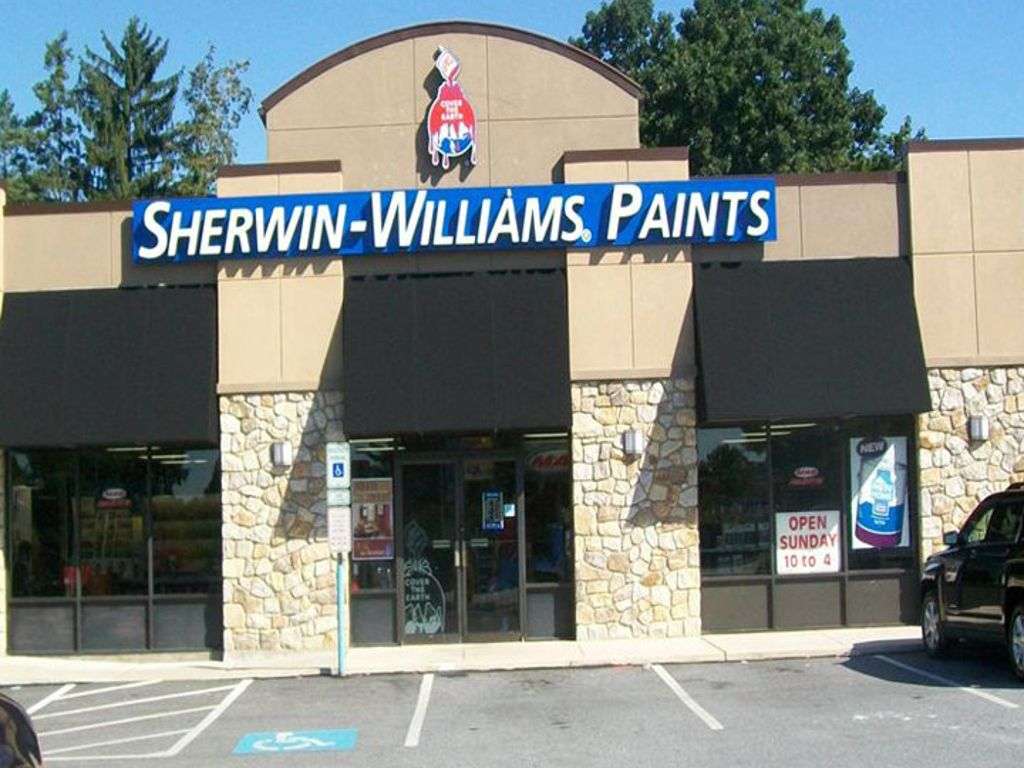This photograph captures the storefront of a Sherwin-Williams Paints store, prominently featuring a blue banner with bold white lettering that reads "Sherwin-Williams Paints." Above this banner, a tilted paint can is depicted dramatically pouring into a large red drop, though the can's lettering is too small to be legible.

At street level, the building is fronted by a series of parking spaces aligned with a horizontal sidewalk. The leftmost space is marked with the blue and white handicap logo, followed by two empty spaces, and a dark-colored vehicle occupies a space just off the right edge of the photograph. 

The upper part of the building showcases a tan facade with darker brown lines accentuating the top edges, leading up to the roof. Behind the Sherwin-Williams banner, the building exterior features beige-colored stone. Flanking the double glass entrance doors are flagstone sections, each mounted with a vertical light fixture at the same height as the door tops.

In the bottom right window, beneath a chocolate brown canopy, a white sign with red lettering announces "Open Sunday 10-4." Adjacent to this sign is a poster displaying an oversized can of paint. A parking sign for the handicap spot is also visible to the left of the doors.